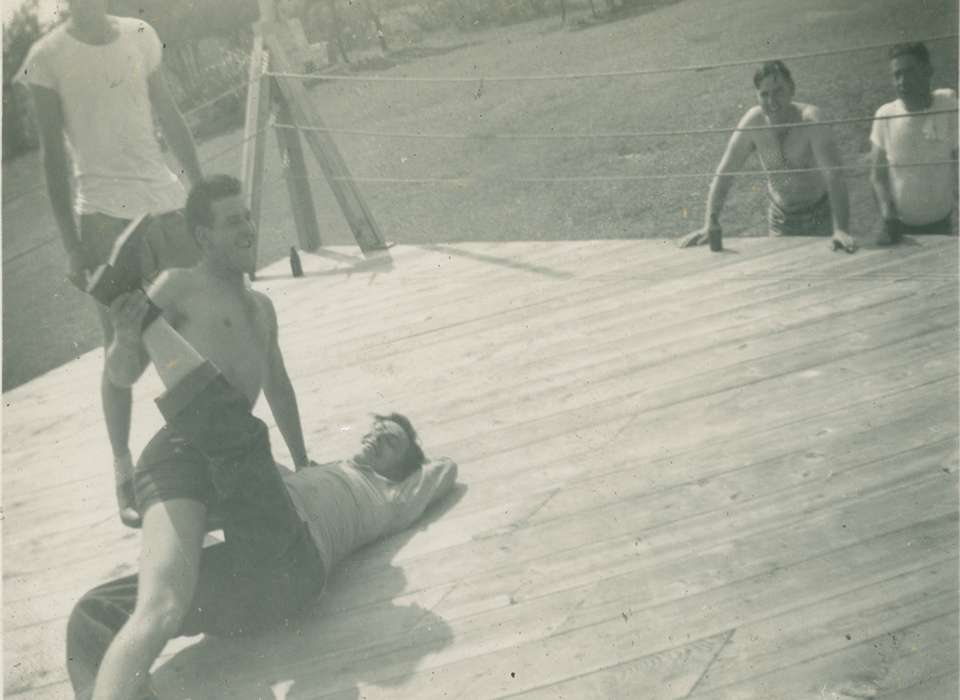The black and white photograph captures a lively scene set outdoors, presumably in a backyard or garden. The focal point is a makeshift wrestling or boxing ring, enclosed by three ropes, where two men are engaged in what appears to be a playful wrestling match. The man on top is shirtless, wearing shorts, and has dark hair, grinning as he pins down his opponent who is dressed in formal attire—shirt, trousers, and shoes—lying on his back with a smile that suggests camaraderie rather than competition. Behind them, a thin man in a white shirt and shorts stands, observing the scene. Outside the ring, two other men, one shirtless and the other in a white shirt, watch with interest. Elements like the grassy surroundings and distant trees add to the casual, impromptu atmosphere of the setting, further indicated by the presence of a beer bottle in one corner of the ring.